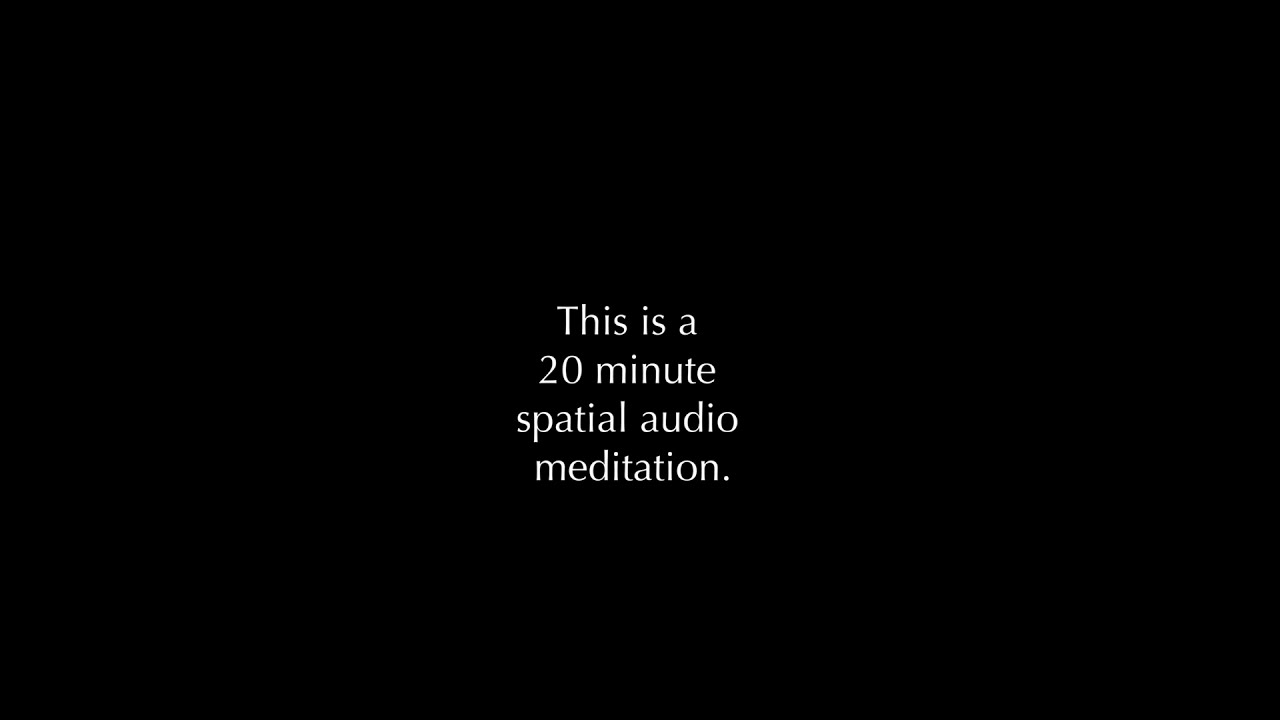The image is a straightforward, minimalistic design featuring a horizontal black rectangle with a single line of white text centered in the frame. The text reads: "This is a 20-minute spatial audio meditation." The font is clear and easily readable, with a period at the end of the sentence. The stark contrast between the white lettering and the black background makes the message stand out distinctly. The simplicity of the image suggests it could have been created using a basic presentation tool like PowerPoint, focusing solely on delivering the message without any additional visuals or distractions. The text is the only content on the screen, emphasizing the message's importance and clarity.